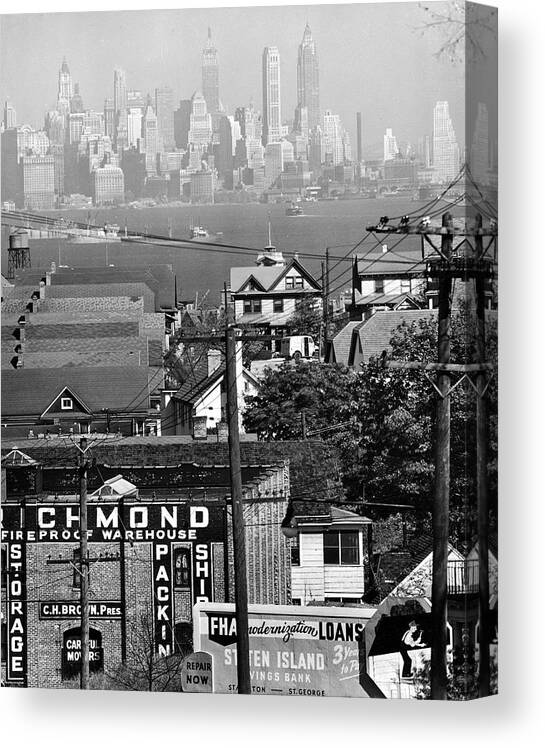This black and white photograph, possibly from the 1930s or 1950s, captures a panoramic view of Staten Island, New York, with significant detail and clarity. The image is rich with elements that tell a story of its era. In the foreground, there's a residential neighborhood with two-story row houses featuring peaked roofs, white exteriors, and gray rooftops. Telephone poles and wires crisscross the scene, adding to the historical ambiance.

Prominently displayed on one of the buildings, likely a commercial establishment, are signs that read "Richmond Fireproof Warehouse," advertising services such as "packing, shipping, storage," and perhaps "repair now." Another building sports a sign for the "Staten Island Savings Bank," mentioning FHA modernization loans. These hints reinforce the image's historical context.

Beyond the residential area, the photograph reveals a body of water, likely the Hudson River or New York Bay, dotted with boats and ferries. This aquatic expanse separates the foreground from the distant city skyline. The skyline itself, shrouded slightly in fog, features iconic skyscrapers that suggest the unmistakable identity of New York City. Notable buildings like the Chrysler Building and possibly the Empire State Building can be discerned, towering among a dense array of tall, slender structures. The composition of the photograph provides a comprehensive and evocative snapshot of urban life, bridging the quaint suburban charm of Staten Island with the bustling, towering grandeur of Manhattan in the background.